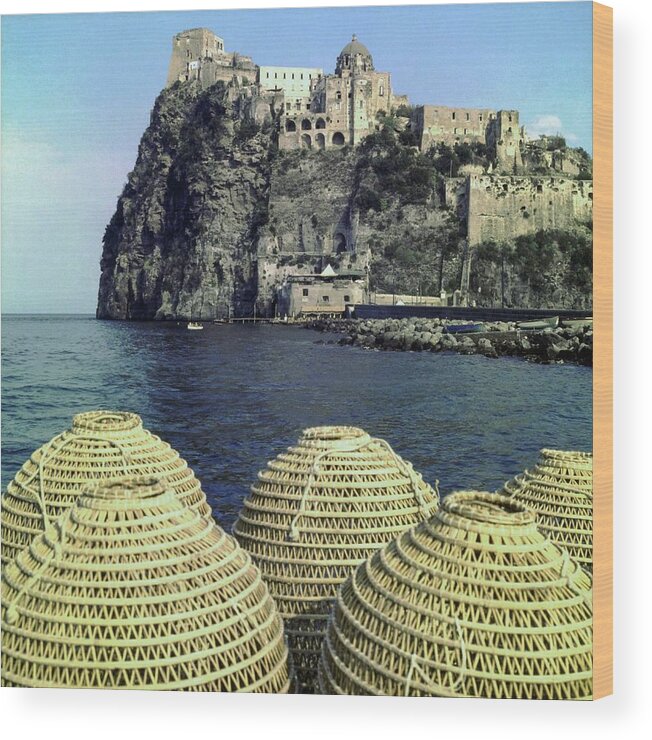The image depicts a charming, albeit slightly faded, postcard from an earlier time. Dominating the scene is an ancient town set dramatically atop a high cliff overlooking a dark, calm ocean. This town features grand stone buildings, including an expansive church or castle-like structure, indicative of its historical significance. Below, closer to the water, there is a jetty extending into the sea, where a small white boat can be seen drifting in the distance. In the foreground, the viewer's attention is drawn to five woven wicker baskets, possibly used for fishing, lined up against the rich, dark stone. The overall palette features a light blue sky that transitions smoothly into the deeper blue of the sea, contrasting with the imposing, weathered stone cliff and its clustered buildings. The intricate details of the scene, from the subtle shades of the sky and water to the textures of the ancient structures and fishing baskets, evoke a serene yet historically rich coastal landscape.